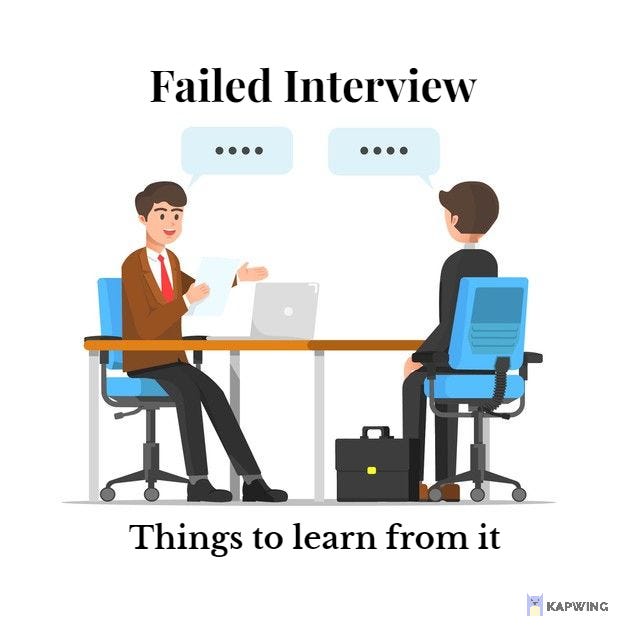This digital infographic employs a cartoon style to illustrate the concept of a failed interview. At the center of the image, two individuals are seated on rolling chairs at a table, seemingly engaged in an interview process. Both figures are dressed in formal suits, highlighting the professional context of their interaction. The person on the left has a laptop open in front of them and is holding a piece of paper, suggesting they may be the interviewer. Above each of their heads, speech bubbles filled with ellipses (three dots) convey an awkward or uncomfortable silence. The top of the infographic is boldly titled "Failed Interview," while the bottom provides a reflective note with the text, "Things to Learn from It," hinting at lessons to be drawn from the depicted scenario.